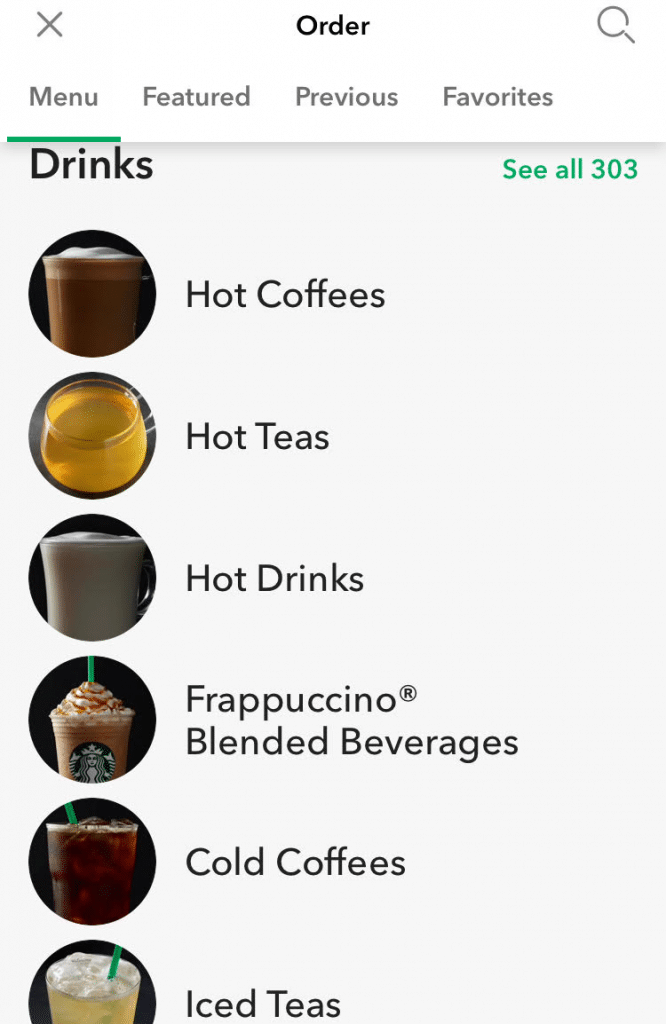This image captures a detailed view of a Starbucks menu interface, showcasing the variety and breadth of drink options available. The screen displays multiple categories of beverages, including hot coffees, hot teas, other hot drinks, Frappuccino blended beverages, cold coffees, and iced teas. Each category is represented by a small image featuring drinks in cups branded with the iconic Starbucks logo. The total number of drink options displayed is 303.

At the top of the screen, the word "Order" indicates that the individual is browsing the digital menu, possibly from a mobile app or website. Adjacent to the menu categories are additional options allowing the user to explore featured drinks, previously ordered drinks, and favorite selections. A search bar, identified by a magnifying glass icon, is located on the right side of the screen, enabling users to quickly find specific items. In the top left corner, a grey 'X' icon provides an option to close the menu interface.